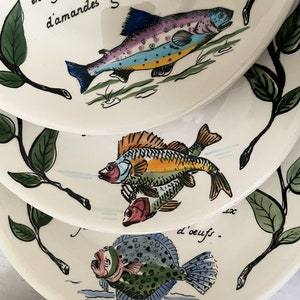This image depicts a set of three circular dishes, which could potentially be coasters. They are partially stacked, displaying about a fourth of each on top of one another. Each dish features a detailed illustration of a fish amidst green leaves framing the image.

The topmost dish showcases a vibrant fish adorned in purple, blue, and yellow hues, facing to the right. Despite some written text being visible, it's unreadable. The middle dish presents two fish, both facing to the left. These fish are characterized by light blue, green, and yellow stripes, with notable fins on their backs and distinct, floppy tails. Finally, the bottom dish highlights a recognizable puffer fish, rounded in shape with a green center, blue outer edges punctuated by black circles, and an open white mouth, also facing to the left.

All three dishes share the common theme of a central fish surrounded by green leaves, reinforcing the cohesiveness of the set.